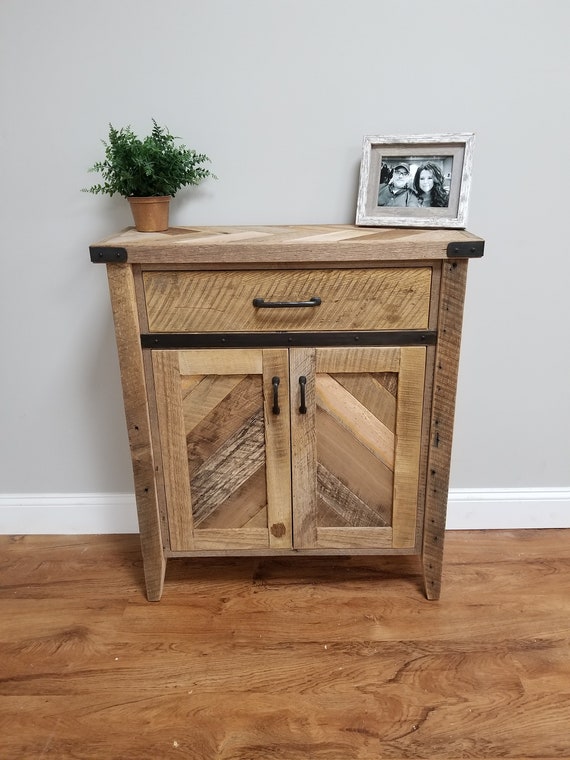This is an indoor color photograph of a handcrafted wooden cabinet standing about three feet tall. The cabinet is positioned against a light gray, almost neutral-toned wall with white baseboards, and it rests on a wooden floor that almost matches its wooden color. The cabinet features two large doors at the bottom, each fitted with black metal handles. The doors are constructed from diagonal wooden panels framed by four wooden frames—two at the sides, one at the top, and one at the bottom. Above these doors is a single pull-out drawer, also adorned with a black handle. The top surface of the cabinet is made of diagonal wooden slabs. Sitting on this surface, towards the left, is a terracotta pot containing a green leafy plant. On the right, there is a white wooden photo frame with a black and white picture of a man and a woman, presumably the owners of the house. The frame has a white matting that contrasts well with the rustic look of the wooden cabinet.